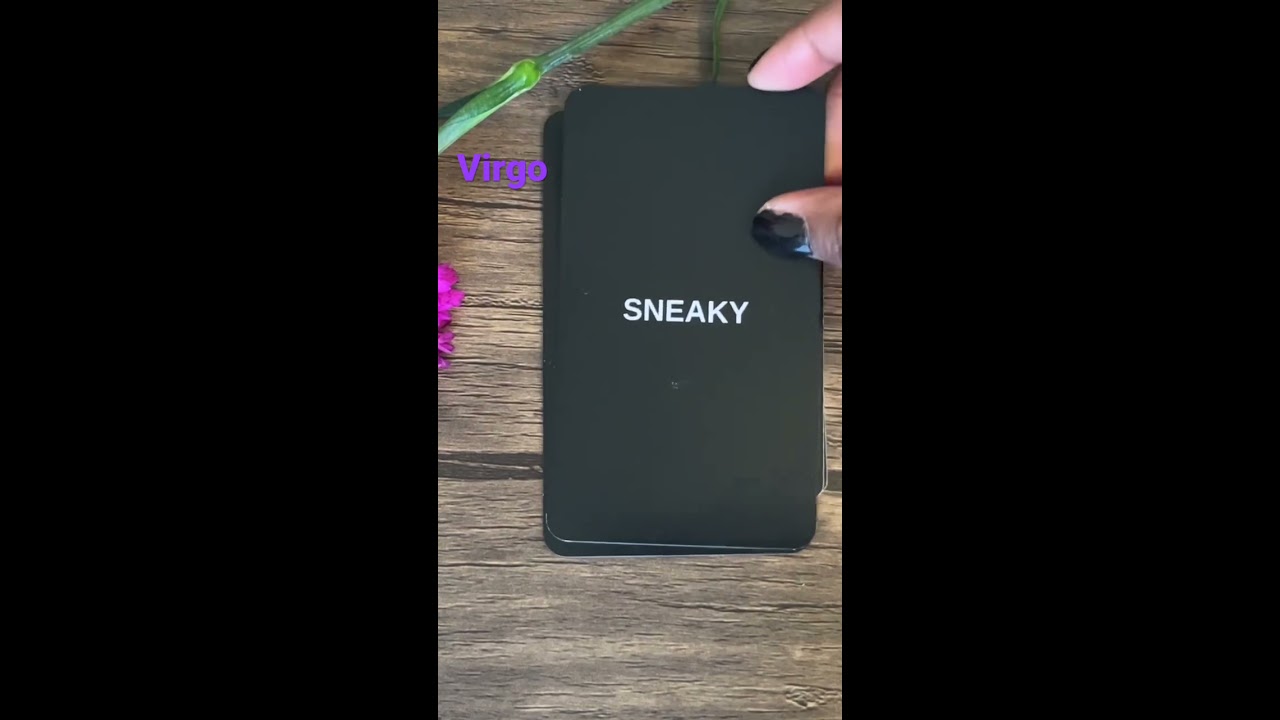In this detailed image, a variety of objects rest on a light brown, weathered wooden surface, perhaps a table or countertop. Central to the composition is a small, black vertical rectangle that might be a card or phone cover. The word "SNEAKY" is prominently displayed in white, all capital letters across the center of this black object. To the left, the text "VIRGO" is inscribed in purple, with only the first letter capitalized, positioned just below the green stem of a partially obscured dark pink flower, possibly a red carnation. A woman's hand, with black-painted nails, delicately grasps the upper right corner of the black object. The overall setting seems to suggest the image could be a screenshot from a mobile device, possibly from platforms like TikTok or Instagram. The color palette includes various shades of brown, black, white, pink, purple, green, and tan, contributing to a visually cohesive and engaging arrangement.